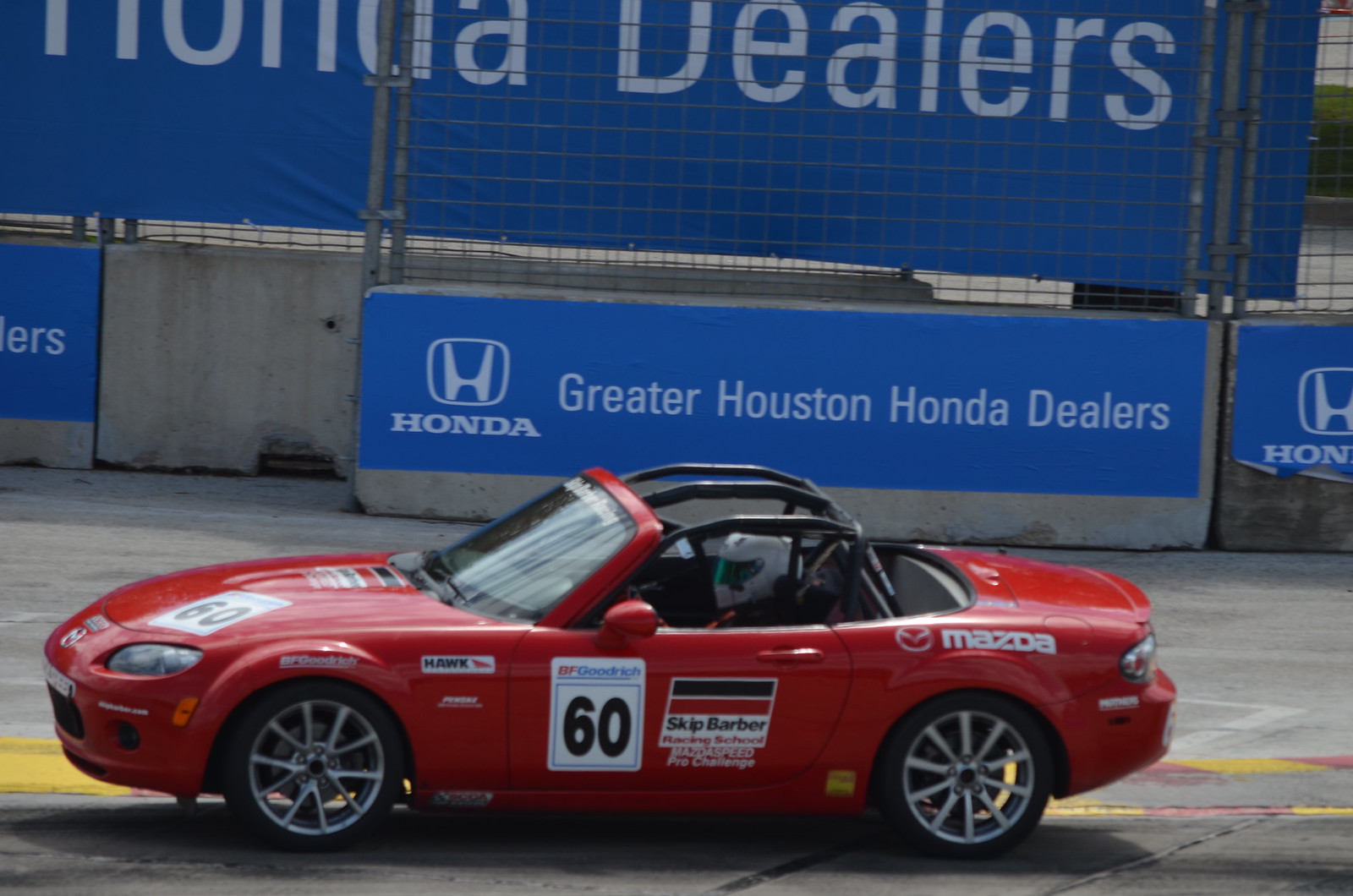This vibrant color photograph, captured outdoors in daylight, features a sleek, red sports car that is both striking and richly detailed. The car, a convertible devoid of a ragtop, boasts prominent safety roll bars over the driver's seat area, emphasizing its racing capabilities. The driver's door carries the name "Skip Barber Racing School," a testament to its high-performance pedigree. Adorned with the number '60' and numerous smaller decals, the vehicle exudes a strong aura of competitive spirit. Above the left rear tire, the name "Mazda" is distinctly visible, adding to its classic appeal. The car is stationary, parked on a concrete surface that suggests a racetrack or parking lot setting. Large concrete barricades in the background bear the branding "Honda" and "Greater Houston Honda Dealers," providing a sense of locality and additional context to the scene.